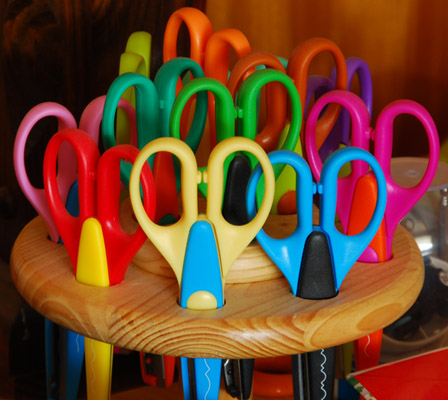The image captures a colorful array of children's crafting scissors neatly arranged in a wooden circular holder, likely a Lazy Susan. Each pair of scissors features unique, serrated edges designed to create various squiggly patterns. The vibrant assortment includes colors such as pink, red, yellow, blue, green, teal, orange, and purple. The wooden holder has individual slots for each scissor, enhancing their accessibility and display. The background reveals some wood paneling and indistinct objects on the right, suggesting a casual, creative setting. Overall, the photo appears to meticulously showcase these artistically functional scissors, possibly for selling or inventory purposes.